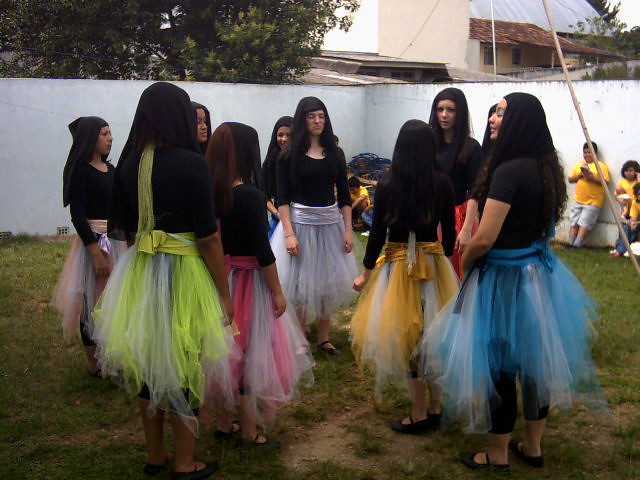In the photograph, a group of women, characterized by their long black hair—some of which appear to be wigs—are standing on grass, donned in an array of dance costumes. All the women wear black tops, which range from long-sleeved to short-sleeved. From their waists, bright, sheer skirts in a multitude of colors flow down, including hues like blue, yellow, pink, and lime green, resembling traditional dance attire. They stand in flat black shoes with a strap across, seemingly prepared to dance. The women are arranged in a circle, suggesting a ceremonial or festive occasion. The setting is outdoors, featuring a white stone wall with spectators leaning against it, observing the scene. To the right, two children in bright yellow t-shirts—one paired with khaki shorts and the other with blue jeans—can be seen. In the backdrop, beyond the white concrete fence and lush greenery, there's a beige concrete building completing the setting.